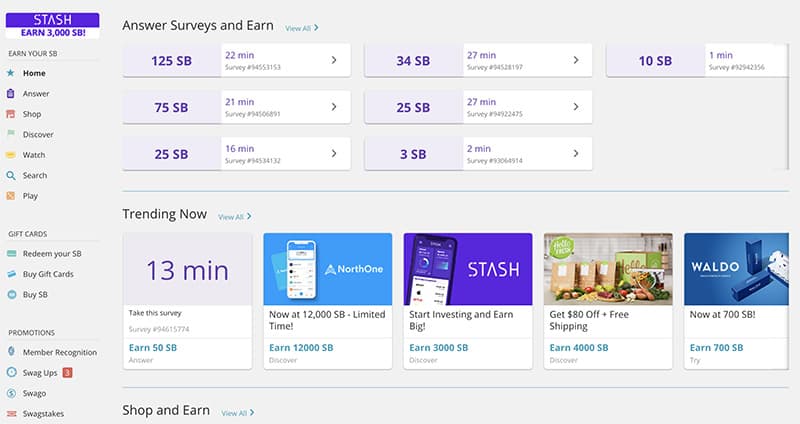The image displays a detailed interface with various sections and categories arranged for user engagement. 

At the top left corner, there's a section titled "Stash," indicating a reward point accumulation titled "Earn 3000SB". Below, there is another header that reads "Earn Your SB", followed by a list of categories: Home, Answer, Shop, Discover, Watch, Search, and Play.

Further down, there's a caption "Gift Cards" with three subcategories beneath it: Redeem Your SB, Buy Gift Cards, and Buy SB. 

In the bottom left, a third main category is labeled "Promotions", which includes subdivisions such as Member Recognition, Swag Ups, Swaggo, and Swag Stakes.

In the center bottom of the image, starting from left to right, there are multiple boxed areas with various images and text:
- The first box has an icon depicting "13min" with the instruction to "Take the survey".
- The second box displays a message: "Now at 12,000SB Limited Time".
- The third box encourages investing, with the text: "Start Investing and Earn Big".
- The fourth box advertises a deal: "Get $80 Off plus Free Shipping".
- The last box mentions another reward opportunity: "Now at 700SB".

Above these boxes are several rectangular boxes featuring different surveys for user participation.